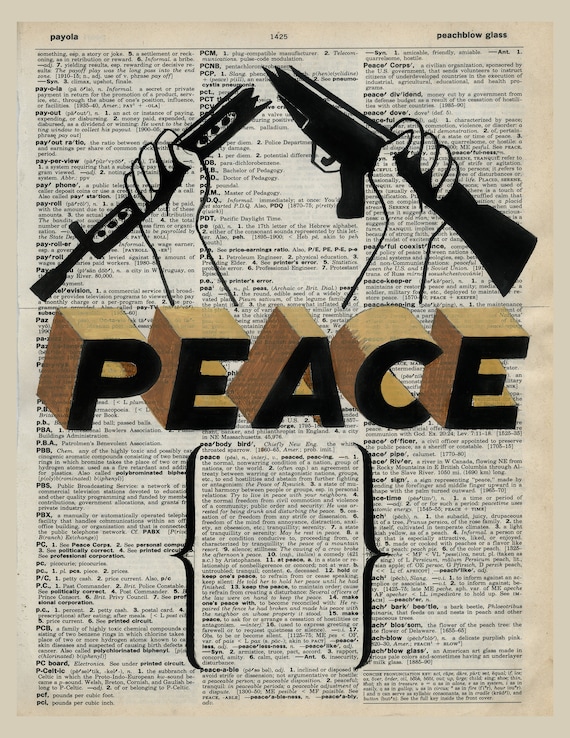The image depicts an aged, possibly yellowing, dictionary page filled with "P" words, including "paola" at the top left corner and "peach glass" to the right of the center page number 1425. Three columns of definitions for various "P" words run down the page. Superimposed on this page are two black-outlined hands, one on the left holding a sword, and the other on the right wielding a bayonet-style gun. The bold, three-dimensional letters of "PEACE" in black-and-wooden hues dominate the middle of the image. Beneath this, a defined black marker outline of the word "peace" completes the scene, intricately filled with the underlying dictionary text.